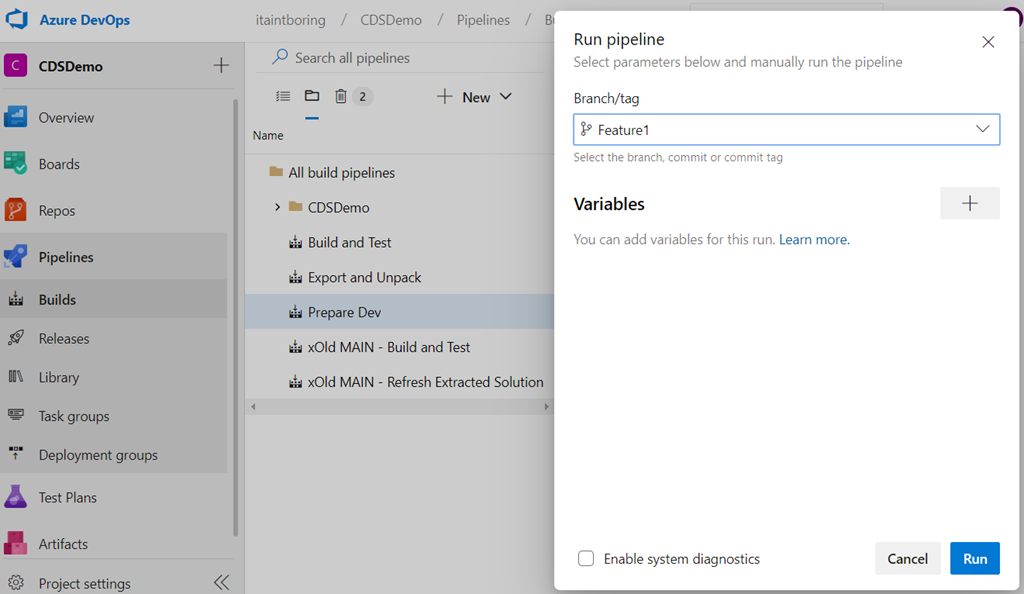This image is a cropped screenshot of an Azure DevOps interface with a visible grayish overlay indicating an active pop-up in the top right corner. The pop-up, titled "Run Pipeline," instructs the user to "Select parameters below and manually run the pipeline." 

The first parameter is labeled "Branch/Tag" on the left, with a drop-down box beneath it displaying "Feature 1" as the selected option. Below this, another section labeled "Variables" appears, with a prompt stating, "You can add variables for this run. Learn more," accompanied by a plus icon for adding new variables. 

At the bottom right of the pop-up, there are two actionable buttons: "Cancel" and "Run." Additionally, off to the right side, an option to "Enable System Diagnostics" is visible, although the full web page on the right is obscured by the pop-up.

In the main Azure DevOps interface, the top left displays the "Azure DevOps" label. Below this, a vertical panel runs along the left side, listing various categories, with "CDS Demo" being the first item. The top header features several categories including "It Ain't Boring," "CDS Demo," and "Pipelines." A search bar labeled "Search All Pipelines" appears beneath these categories, followed by columns titled "Name" and "Folders." The primary folder displayed is "All Build Pipelines."